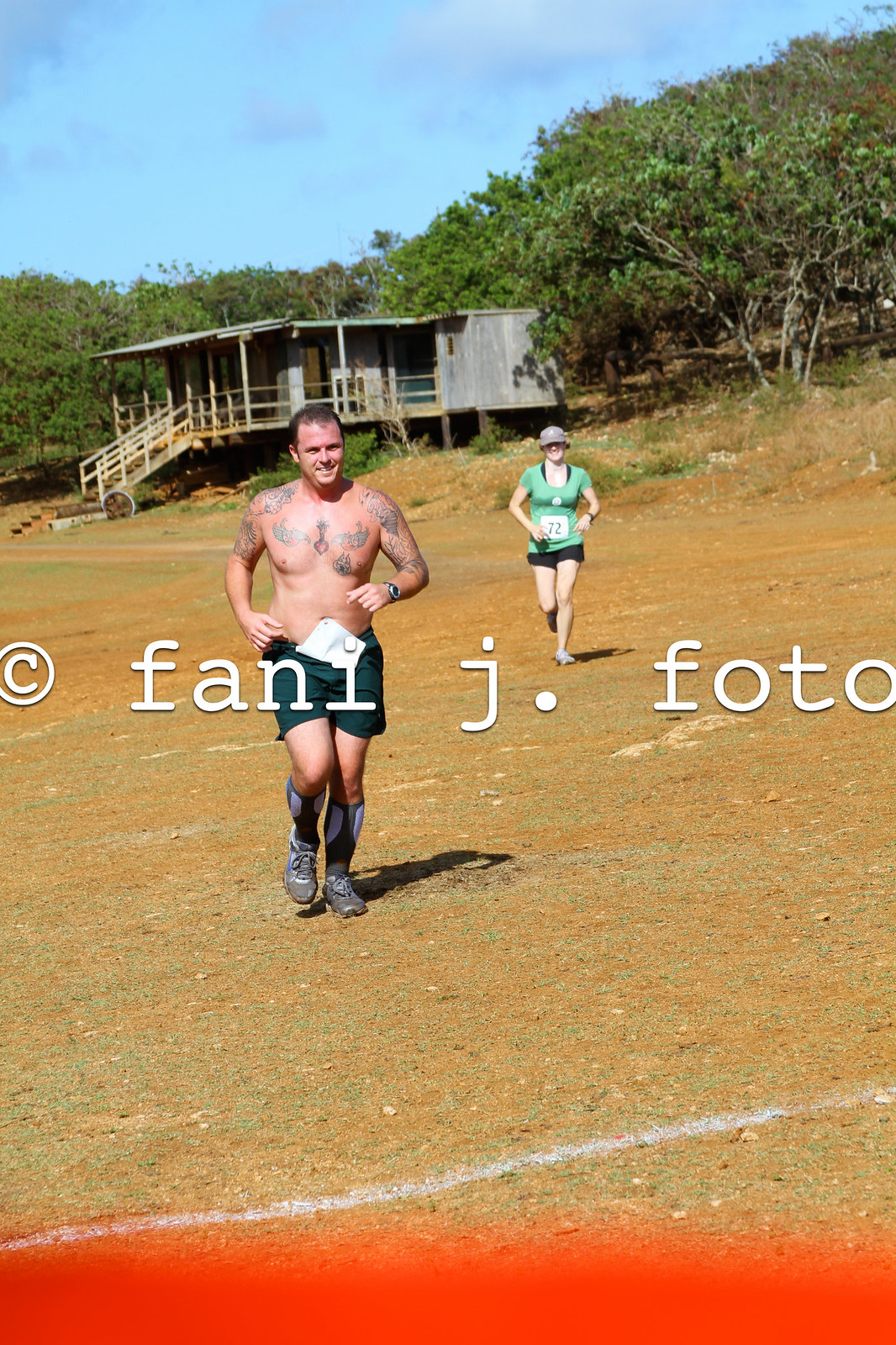In this vibrant photo set on a dusty, dry field with lines resembling a playing field's end zone, two people are captured jogging towards the camera. A muscular, shirtless man in black athletic shorts, gray running shoes, and sporting tattoos and a watch on his left wrist, runs in the foreground. His shorts partially cover a numbered bib. Behind him, about 12 feet back to his right, a woman in a light green shirt, black shorts, and a hat is also jogging. She wears the number 72 and is seen smiling. The scene is lit by bright sunlight, accentuating their brisk activity. In the background, a wooden cabin with a walkway leading to the field and a wooden railing stands amidst some green trees against a blue sky. An overlay of text displaying "© Fanny J. Foto" spans across the middle of the image, and a red bar is noticeable at the bottom, possibly as part of the photo's design.